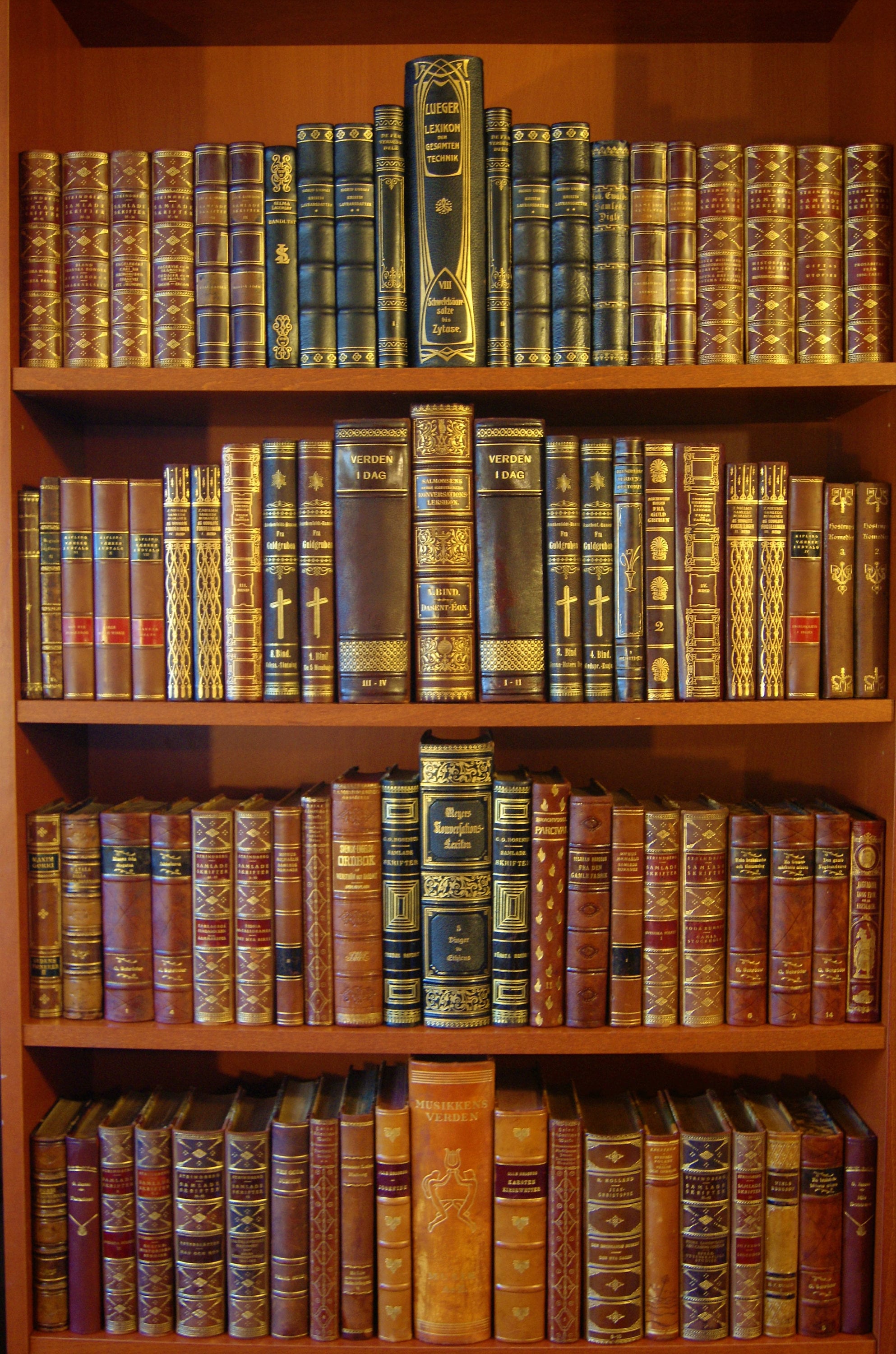This close-up image showcases a large, antique wooden bookshelf with four thin shelves, filled to the brim with volumes of books arranged with meticulous care. The bookshelf, crafted from dark brown wood, holds books aligned by color and size to create a visually appealing pattern. Each shelf features a central taller book flanked by two slightly shorter books, giving the appearance of a triangle tapering off towards the ends. The spines of the books are in various shades of maroon, dark brown, black, and orange, often with gold accents and intricate designs like crosses, geometrical shapes, and scrolls, suggesting religious or historical content. The books are predominantly hardbacks, with leather-like covers, some appearing to be part of matching sets. The arrangement and patina of the bindings give the entire bookshelf an old-fashioned, elegant look, reminiscent of a meticulously curated collection of antique volumes.